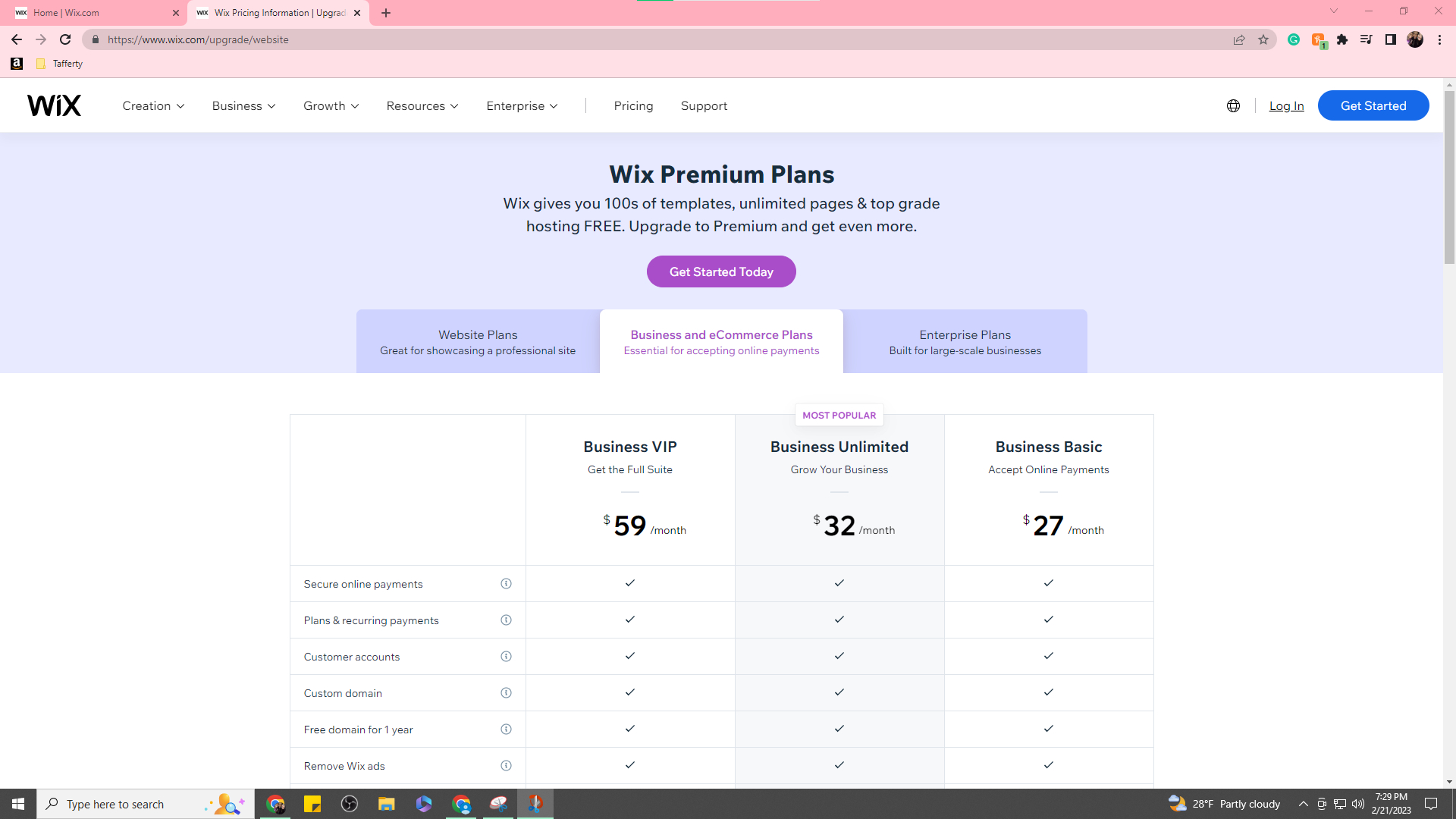A detailed browser window screenshot displaying the Wix.com upgrade page is shown. At the top, the browser interface includes navigation elements such as a left arrow, right arrow, and refresh button. The URL bar highlights the address: [www.wix.com/upgrade/website](http://www.wix.com/upgrade/website), with the page title indicating "Wix Pricing Information".

The page content is focused on various Wix premium plans and their respective features. At the center, there are headings and information blocks detailing different types of plans such as "Website Plans", "Business and E-commerce Plans", and "Enterprise Plans." Each section emphasizes key benefits like hundreds of templates, 11 pages, top-grade hosting, and features like secure online payments.

A column on the right side elaborates on specific pricing tiers:
- Business VIP: $59/month
- Business Unlimited: $32/month
- Business Basic: $27/month 

The price column further highlights benefits such as a custom domain free for one year, recurring payments options, and access to the Wix app.

Accessory icons on the screen indicate the use of other applications such as Grammarly, Google Chrome, Notepad, and OBS. The system tray shows current weather conditions with an icon of clouds in front of a moon, indicating 28 degrees Fahrenheit and a description "partly cloudy". The timestamp reads 7:29 PM with date details "02/06/21".

This comprehensive snapshot captures both the browser interface and detailed web page content, providing a clear overview of the Wix upgrade options available.